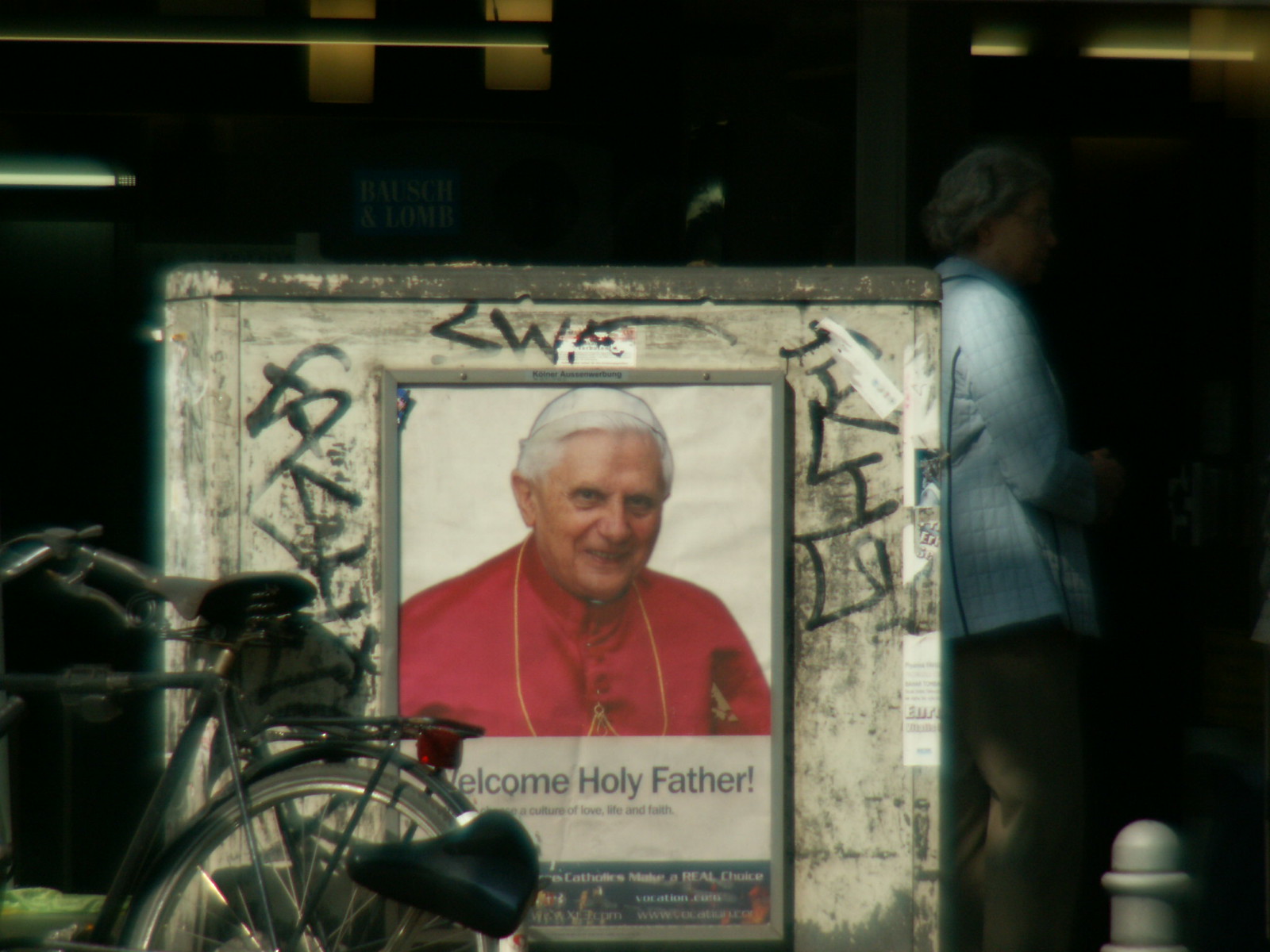The image depicts a white, mottled, square concrete utility box situated outdoors, likely on a city street. The box is covered in black graffiti and appears dingy. At its center, a large poster of Pope Benedict is prominently displayed. The Pope, clad in a white skull cap and a red silk robe with gold lining, looks thoughtfully off to the right. The poster reads, "Welcome, Holy Father," with additional, smaller text beneath. Leaning against the left side of the utility box is a black bicycle. In the background, a woman's white quilted winter coat and the faint Bosch and Lomb logo, partially shadowed, can be discerned against an otherwise dark backdrop. The scene suggests a bustling urban environment despite the obscured surroundings.